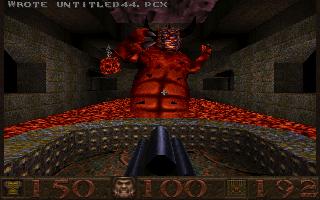This screenshot captures a vintage video game from the 90s or early 2000s, displaying a first-person view inside a dark, gray brick dungeon. Dominating the scene is a towering, monster-like red creature, seemingly a boss character, surrounded by lava. The creature, with claws for hands, appears to be holding a lantern in its left hand. In front of this menacing figure is a weapon, possibly gun-like, suggesting the perspective of the player ready to engage the enemy. The bottom of the screen features a dark brown banner with game stats: a gold “150” near a crown logo, followed by a face icon displaying “100,” and another emblem marked "192." The ceiling is brown, and the overall ambiance emphasizes the classic, challenging nature of old-school gaming, made dramatic by the red background and the squarish, arm-like structures protruding from the monster.